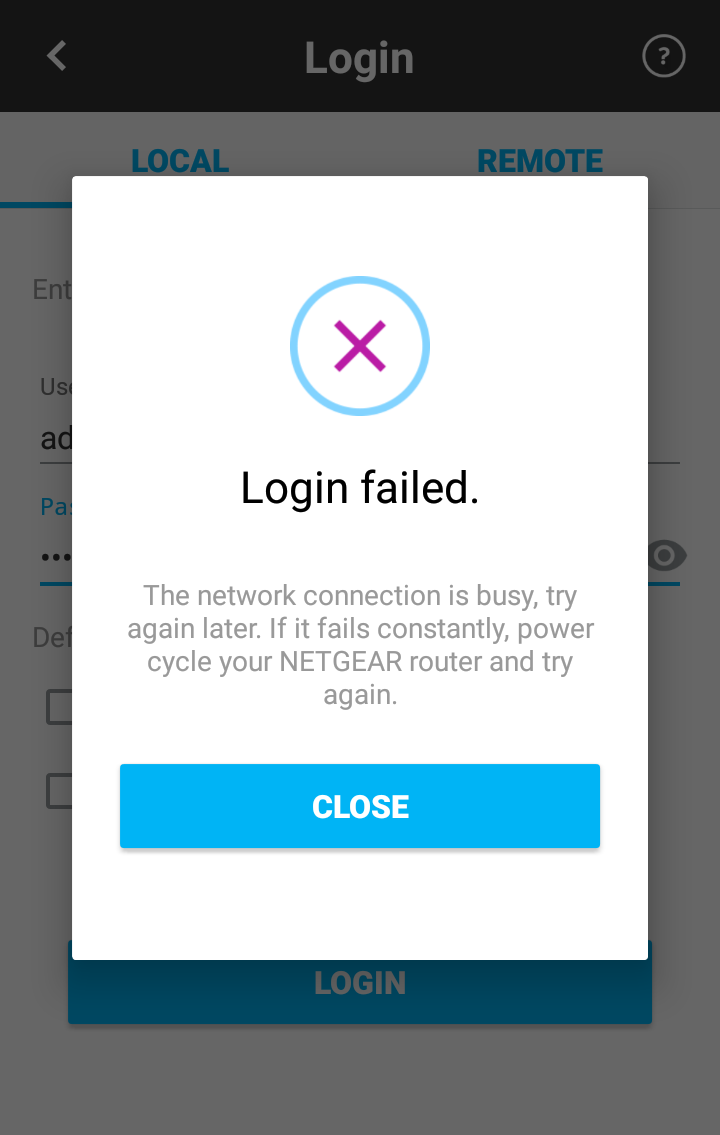The image depicts a rectangular white pop-up box displaying a notification with the title "Login Failed" in bold, blue text. Within the white box, there is a blue outline of a circle containing a purple "X". Below the title, the message reads: "The network connection is busy. Try again later. If it fails constantly, power cycle your Netgear router and try again." At the bottom of the pop-up, there is a blue button labeled "Close."

The background, partially obscured by the pop-up, appears to be a darkened webpage or application interface. The top section of this interface features a dark bar with a white leftward-pointing arrow, followed by the text "Login." To the right, there is a question mark icon encased in a circle, suggesting help or information. Below this, labels reading "Local" and "Remote" are visible.

Underneath the pop-up, there are additional elements that are not fully discernible due to the overlay. These include truncated text starting with "ENT," a username field with some text, and a password field represented by obscured dots. Another partial text "DEF," possibly a truncated word, is also visible. Towards the bottom of the obscured interface, there is a prominent blue "Login" button. The overall scene conveys a user interface where an attempt to log in has failed due to a network connectivity issue.